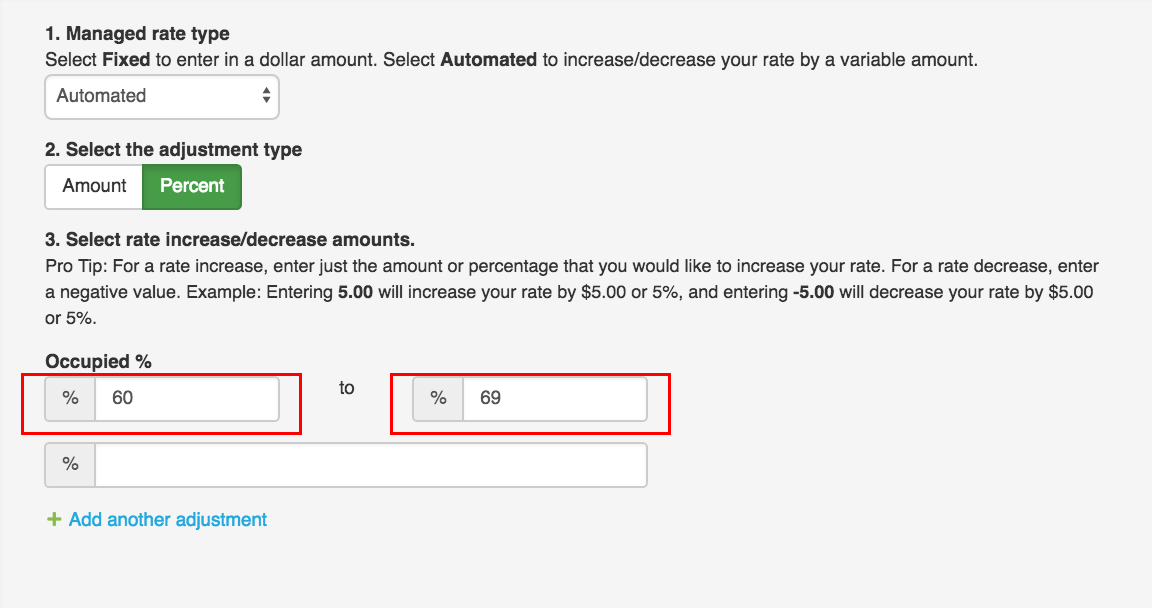The screen features a light gray background with black text, organized into three numbered items. The text provides detailed instructions for managing rate types, selecting adjustment types, and specifying rate increase or decrease amounts.

1. **Managed Rate Type:** This section instructs users to choose between 'Fixed' and 'Automated' options. 'Fixed' allows entering a specific dollar amount, while 'Automated' varies the rate based on set parameters. A dropdown menu with up and down arrows currently displays 'Automated'.

2. **Select the Adjustment Type:** This part of the screen offers two side-by-side selection rectangles. The first rectangle is white and labeled 'Amount', and the second is green and labeled 'Percent', allowing users to specify the nature of their rate adjustment.

3. **Select Rate Increase/Decrease Amounts:** This section provides a "Pro tip" advising users on how to input values for rate changes. For an increase, users should enter the desired amount or percentage of the increase. For a decrease, a negative value should be used. An example clarifies that inputting "$5" will increase the rate by $5 or 5%, while entering "-$5.00" will decrease the rate by $5 or 5%. Below this explanation, two input boxes are present beneath the label 'Occupied Percent', each highlighted with a thin red line.